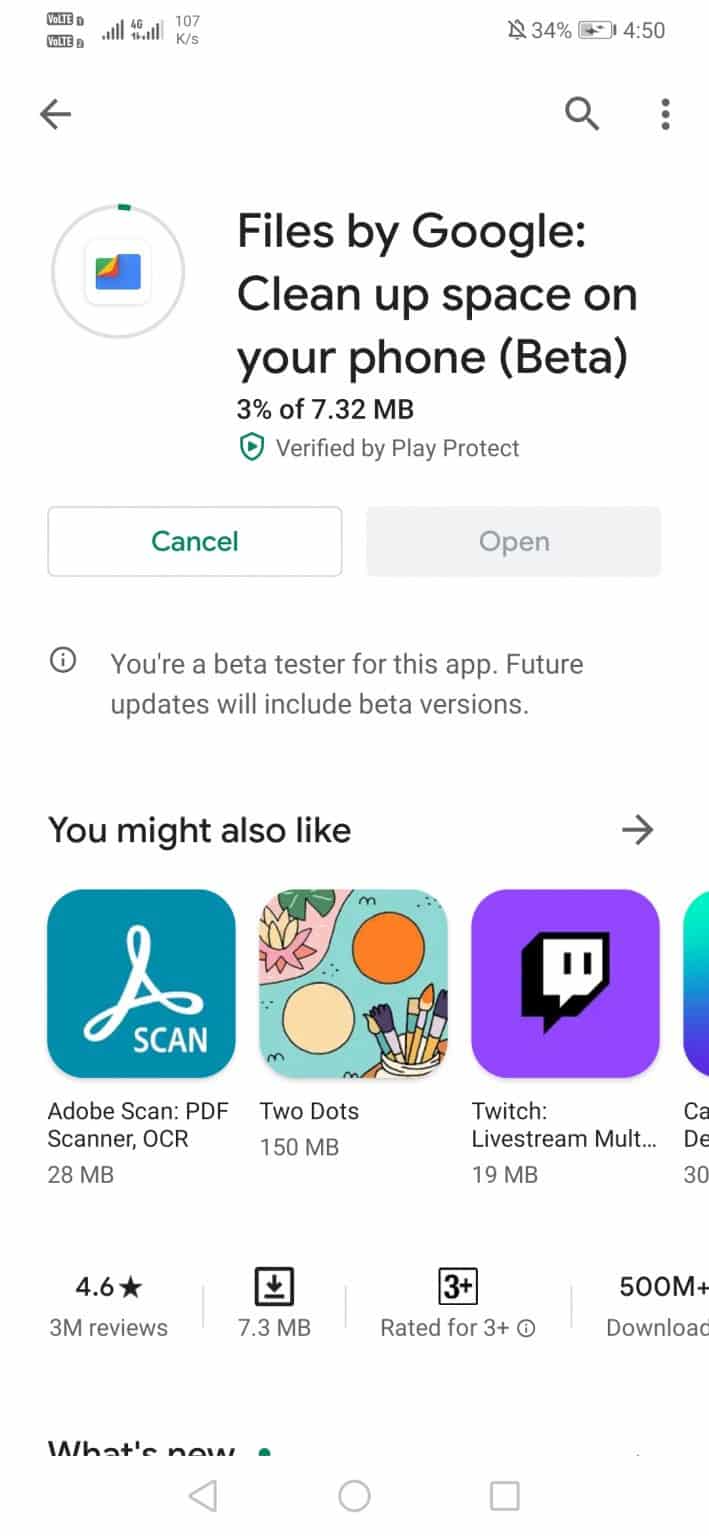Screenshot Description of the "Files by Google" App Interface:

**Top Section:**
- **Upper Left Corner:** Cellular signal data icon.
- **Upper Right Corner:** Silent mode icon (bell with a line through it), 34% battery life indicator, and the time displayed as 4:50.

**Below the Status Bar:**
- **Horizontal Toolbar:**
  - **Left Side:** Back arrow icon.
  - **Right Side:** Magnifying glass (search) icon followed by a three-dot menu icon.

**Main Content Area:**
- **Header:** "Files by Google - Cleanup space on your phone" with "Beta" in parentheses.
- **Progress Indicator:**
  - Text showing "3% of 7.32 MB Verified by Play Protect."
  - To the left of the text, a green shield icon with a play button inside.
  - To the left of this icon, a circular progress indicator (approximately 5% filled) featuring a square with a blue paper motif.

**Action Buttons:**
- Two buttons labeled "Cancel" and "Open."

**Information Section:**
- An 'i' (information) icon followed by the text: "You are a beta tester for this app. Future updates will include beta versions."

**Recommendations Section:**
- Heading: "You might also like" with an arrow icon.
- List of three suggested apps:
  - **Adobe Scan**
  - **Two Dots**
  - **Twitch** (with a purple background and a chat bubble with eyes icon)
- **App Details (for Twitch):**
  - 4.6-star rating
  - 7.3 MB size
  - Rated for ages 3+
  - 500 million downloads
  - "What's new" section (cut off by the edge).

**Bottom Section:**
- Standard Android UI navigation buttons.